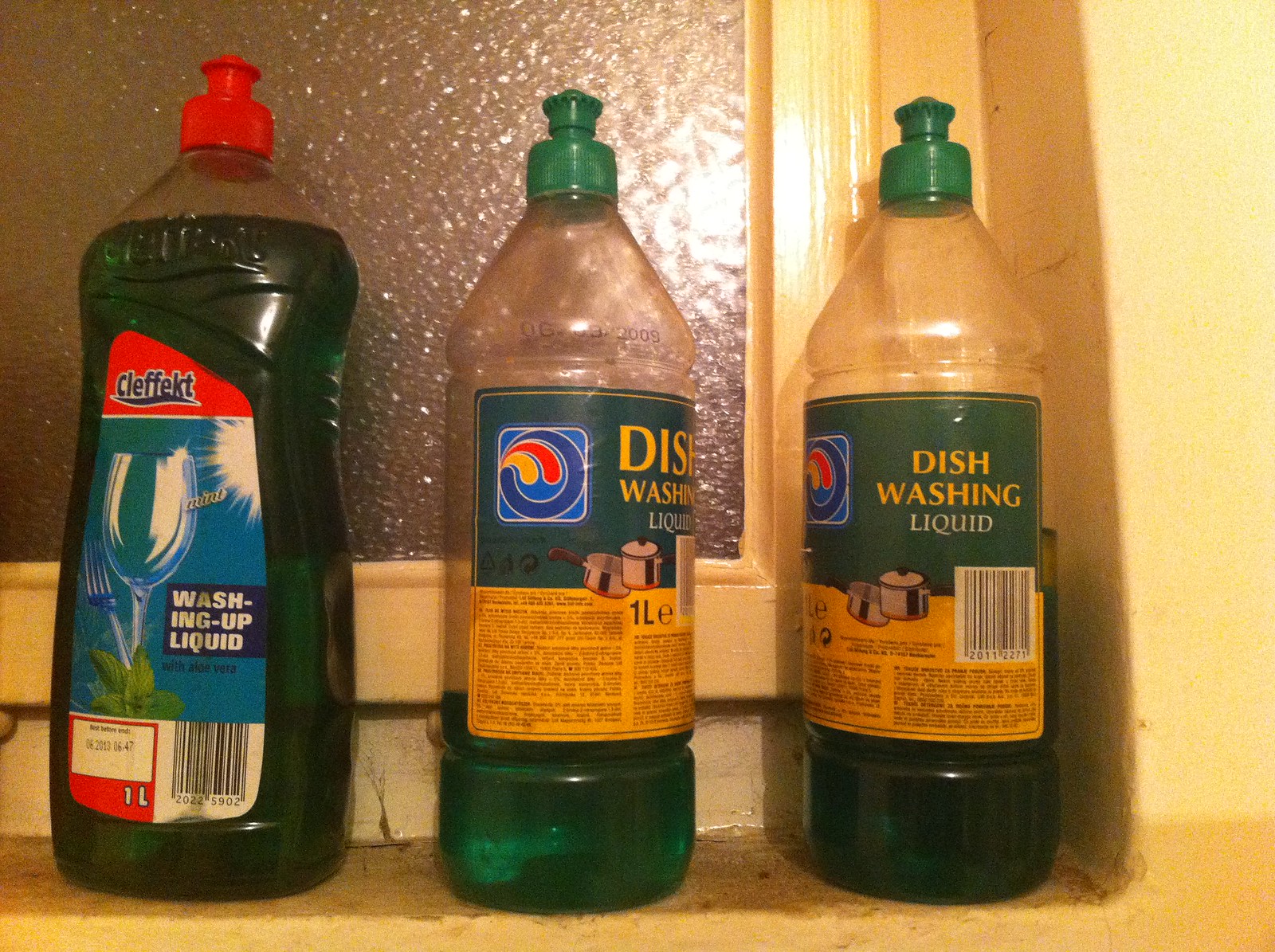The photograph depicts three plastic bottles of dishwashing liquid positioned on the windowsill of a small indoor alcove. The central and right bottles are of the same brand, both featuring green nozzles and labels with a green upper half and a yellow lower half, inscribed with the words "DISHWASHING LIQUID." These two bottles are not completely filled, containing dark green soap. The bottle on the left contrasts with a taller frame, a bright red cap, and is distinctly labeled “CLEFFECT” with an image of a sparkling clean wine glass. The liquid in the Kleffect bottle is also dark green but it is almost full. The setting features a yellow window frame and bright yellow walls, with a mustard yellow shelf. The window glass has a privacy texture that allows light to pass through but obstructs clear visibility. This image captures the simplicity of the indoor setting with flash photography, highlighting the varying heights, brands, cap colors, and liquid levels of the dishwashing bottles.